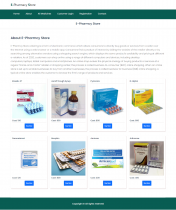The image depicts a cluttered and unclear interface. At the top and bottom, there are green bars that frame the content, although the text within these bars is unreadable due to the blurriness. In the center, there are various categories listed that users can presumably click on, but this text is also indistinct. To the left, near the top, additional text is visible, followed by bold text that introduces a paragraph below it. Unfortunately, the paragraph's content is also obscured. The main focus of the image appears to be a collection of eight images showing boxes and bottles, likely of medication or supplements, in various colors including blue, red, and yellow. These products seem to be accompanied by pricing information, but the details remain indiscernible. The overall visual impression is one of a disorganized and difficult-to-navigate layout.